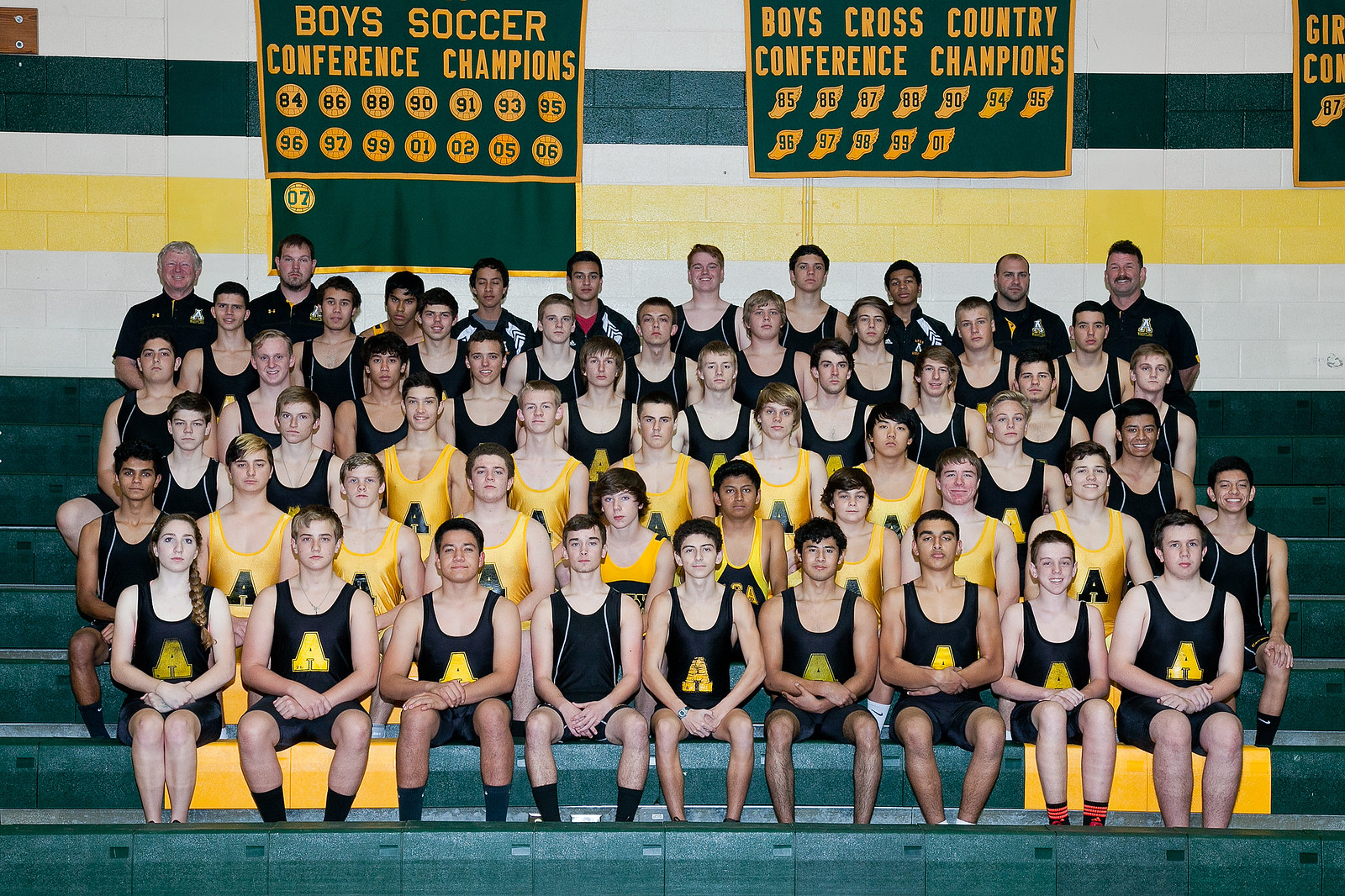The photograph captures a vibrant scene inside a gymnasium where approximately 50 young men and a few adults are gathered and posed on tiered, dark teal bleachers. The majority of the group, presumably aged around 14 to 15 years old, are uniformly dressed, with some wearing black tank tops featuring a large yellow letter "A," while others sport yellow tops. In the front row to the far right, there's a girl with long hair braided into a ponytail, a notable exception in the predominantly male group. High on the bleachers, to the far left and right, stand a couple of elderly men, likely in their 40s or 50s, who appear to be coaches. The backdrop consists of a wall adorned with black and yellow striped decorations, along with several banners proclaiming achievements in boys' soccer and cross-country, such as "Boys Soccer Conference Champions" and "Boys Cross-Country Conference Champions," celebrating their competitive victories.